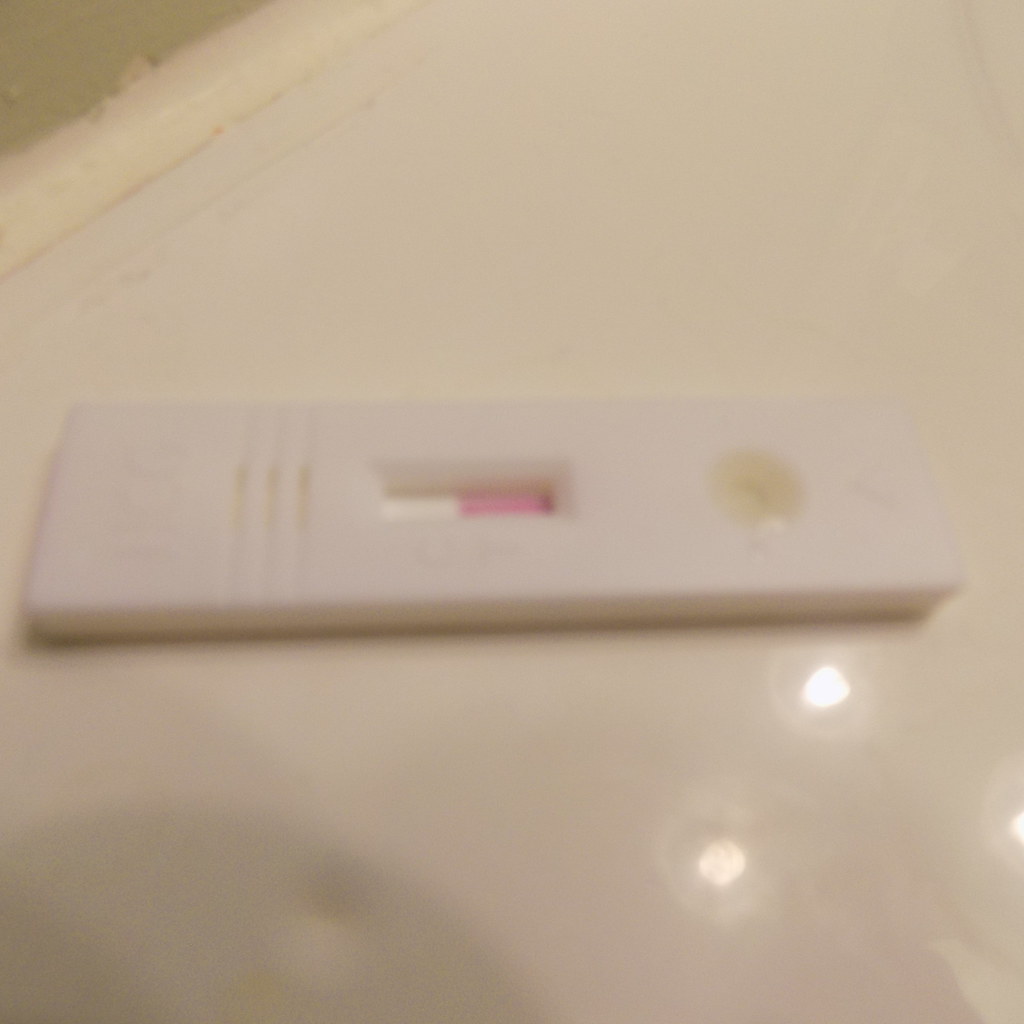This image, albeit blurry, depicts a close-up view of a testing kit, potentially a COVID-19 or pregnancy test. The object, rectangular in shape, is positioned on a white, reflective surface that catches light from three distinct sources. The testing kit features three indentations: a larger one in the center housing the indicator, which displays a dual-colored result—half white and half pink. To the right, there's a small circle veiled under a yellow-tinted plastic film, presumably the sample application area, marked by an indented triangle pointing towards it. Although the text on the left side of the kit is unreadable due to the blur and poor lighting, a round shadow is noticeable at the bottom left corner of the image. The overall lighting is dim, contributing to the lack of clarity.